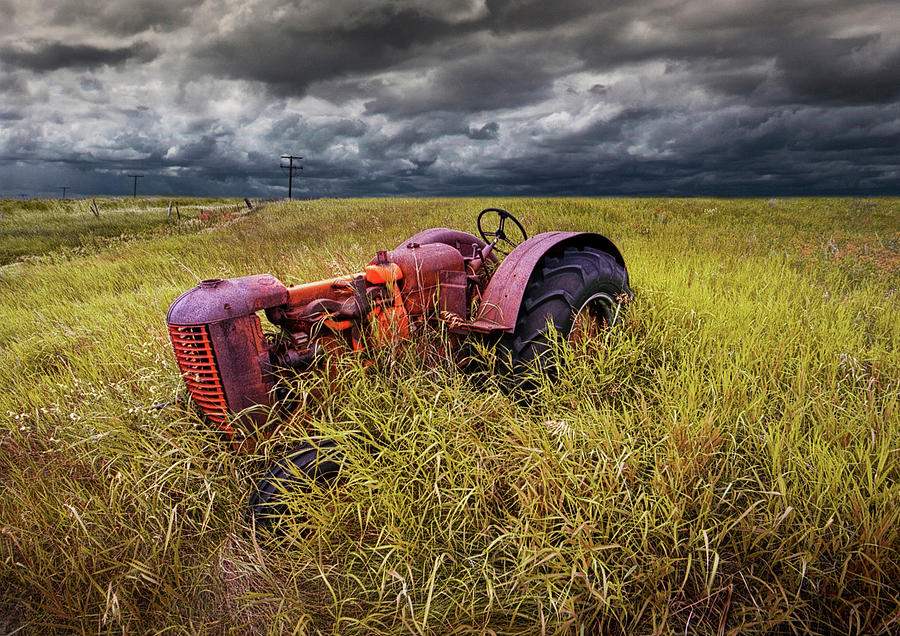The outdoor photograph captures a dramatic scene with a dark, stormy sky filled with ominous clouds, highlighted by patches of white. Below this turbulent sky lies a vast field of tall, yellowish-green grass that hints at the change of seasons. In the middle of this natural expanse stands an old, abandoned tractor. The tractor boasts a tired, brick-red body, accentuated by a neon orange front grill and tinged with spots of rust, indicating years of disuse. The back left tire of the tractor seems partially buried in the long grass, further suggesting its long-term abandonment. A black steering wheel is visible from this angle, as well as a large, worn black wheel. Positioned slightly to the right, the tractor faces away from the viewer, adding a sense of mystery to its story. In the background, power lines can be seen against the dramatic sky, adding a subtle reminder of distant civilization to this otherwise forgotten scene.